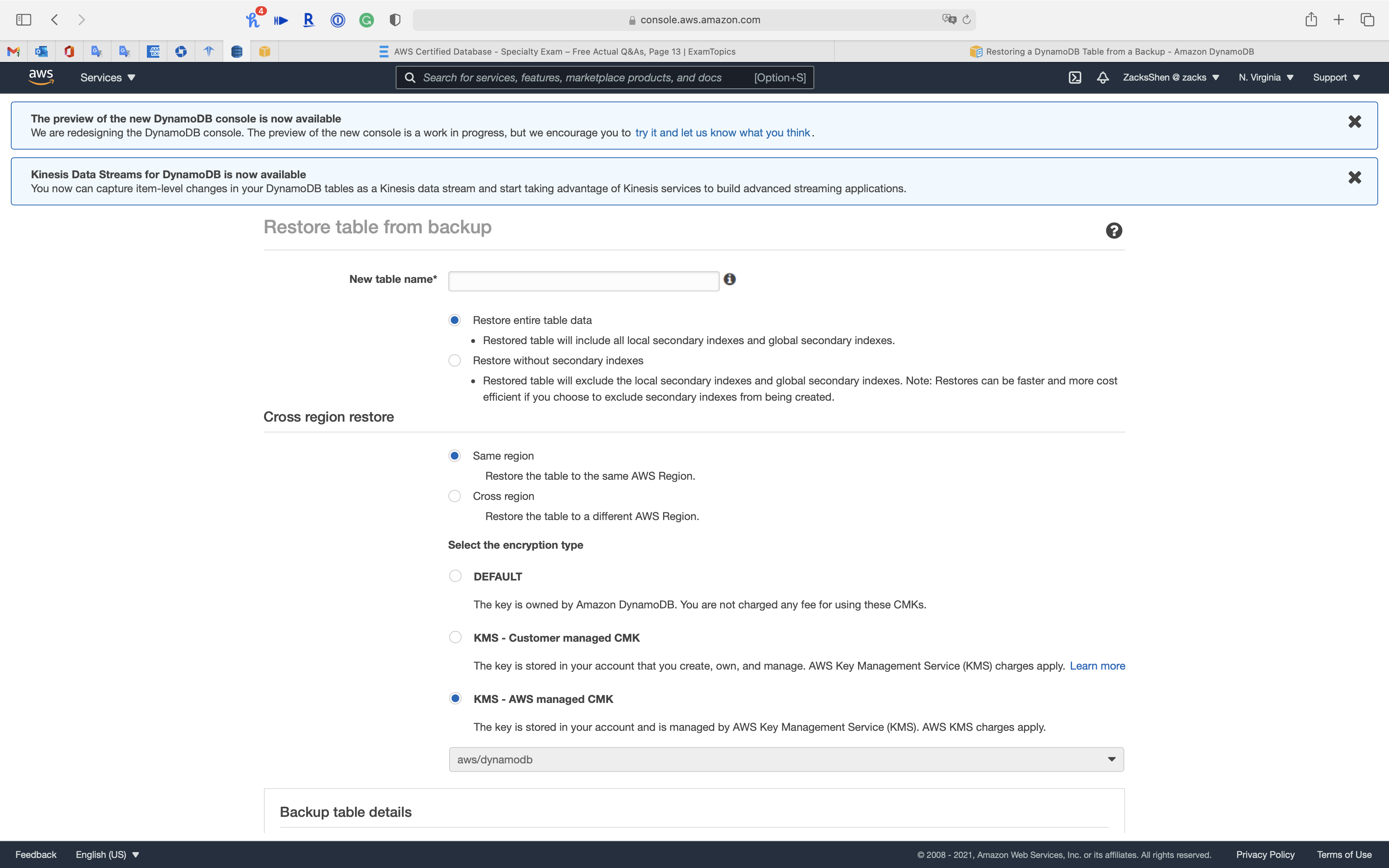A screenshot of a computer screen displaying a webpage related to Amazon.com. At the top of the screen, there is a navigation bar with icons for various applications including Gmail and Internet Explorer. Below this, a black bar with the AWS (Amazon Web Services) logo is visible, followed by a few blue information strips. The first blue strip announces the availability of the new Dynamic OB Console preview, encouraging users to test it and provide feedback. Another strip mentions the availability of "Kinesis Data Streams for DynamoDB". 

The main content of the screenshot focuses on a feature allowing users to restore a table from a backup. The interface prompts the user to enter a new table name and specifies that the option to restore all table data has been selected. Additionally, the option for a cross-region restore is set to the same region. The user can select the encryption type, with the KMS AWS-managed encryption selected in this case. Above this section, drop-down menus are available for further configuration of the table details.